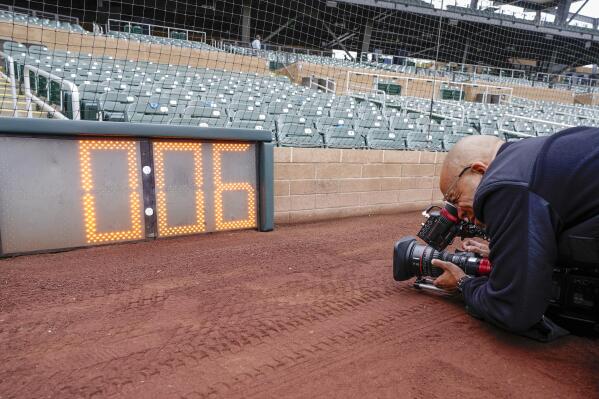In the image, set in an empty baseball stadium, a light-skinned, balding African-American man is the focal point. He is wearing a blue jacket and glasses, and he is positioned on the ground to the right, intensely focused on capturing a shot with his commercial-grade camera, equipped with a square filter and a large lens. The man is squinting as he aims at a digital sign with the number "006" displayed in an orange dotted pattern, propped against a tan brick retaining wall. The ground he is on is a reddish-brown dirt path, marked by visible tire tracks. Rising behind him are rows of empty, light green bleacher-style seats that ascend stadium-like into the background. A net extends upward, likely behind home plate, reinforcing the baseball stadium setting. The photo captures the quiet, anticipatory atmosphere of the scene, devoid of any spectators.